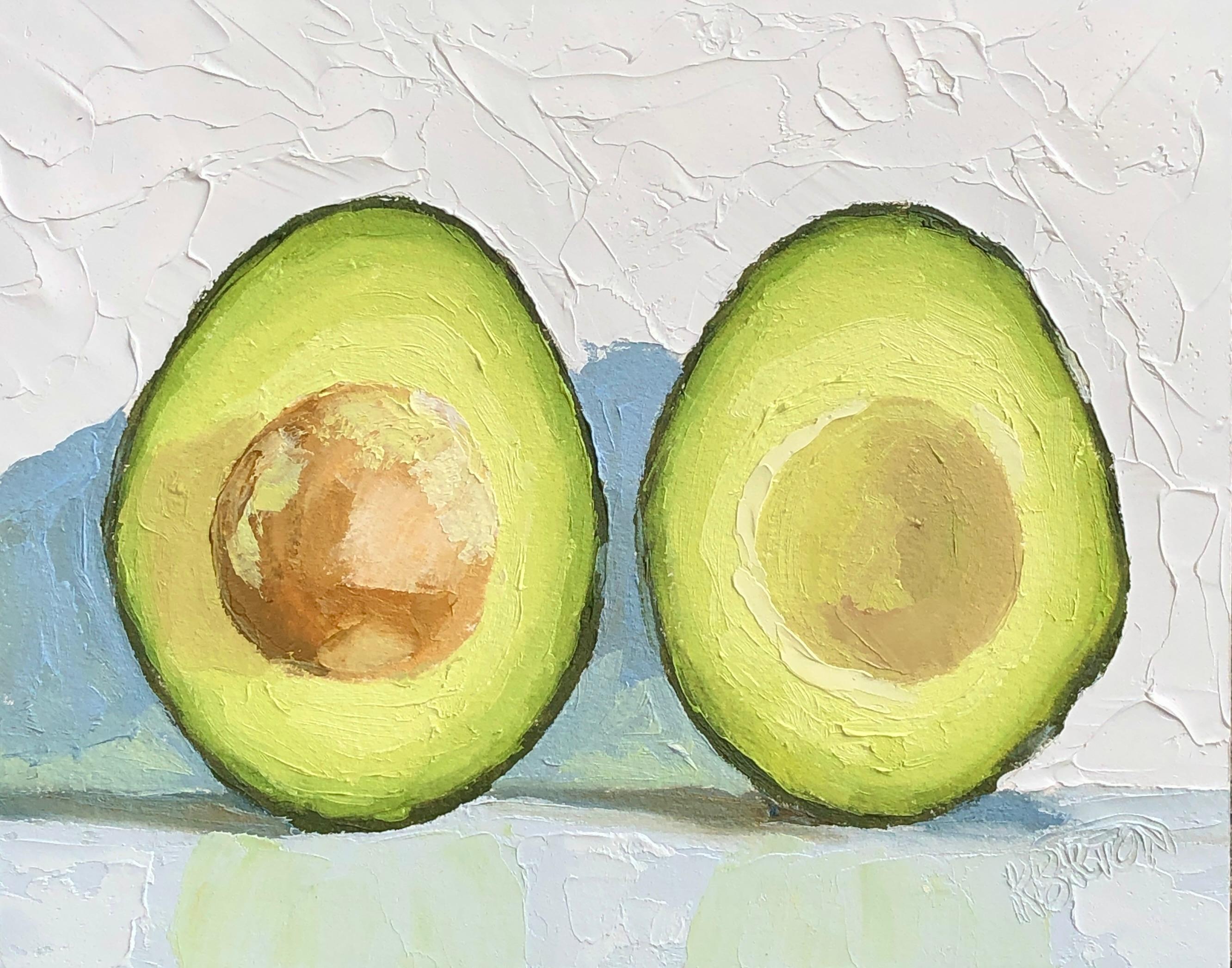The oil painting depicts a cut-in-half avocado placed on a light blue tabletop. The left half of the avocado prominently features the large pit, rendered in various shades of brown with hints of green, while the right half showcases the negative space where the seed once was. The avocados are vibrantly colored, with a dark green outer skin transitioning to lighter greens and almost yellow hues towards the center. Visible brush strokes lend the painting a textured appearance, particularly noticeable in the spackled white and blue-shadowed background. Green reflections and subtle dark grey shadows are visible around the avocados on the tabletop, enhancing the realistic effect. A signature attributed to either R. Bracken or Kay Barton is inscribed on the lower right side of the artwork.